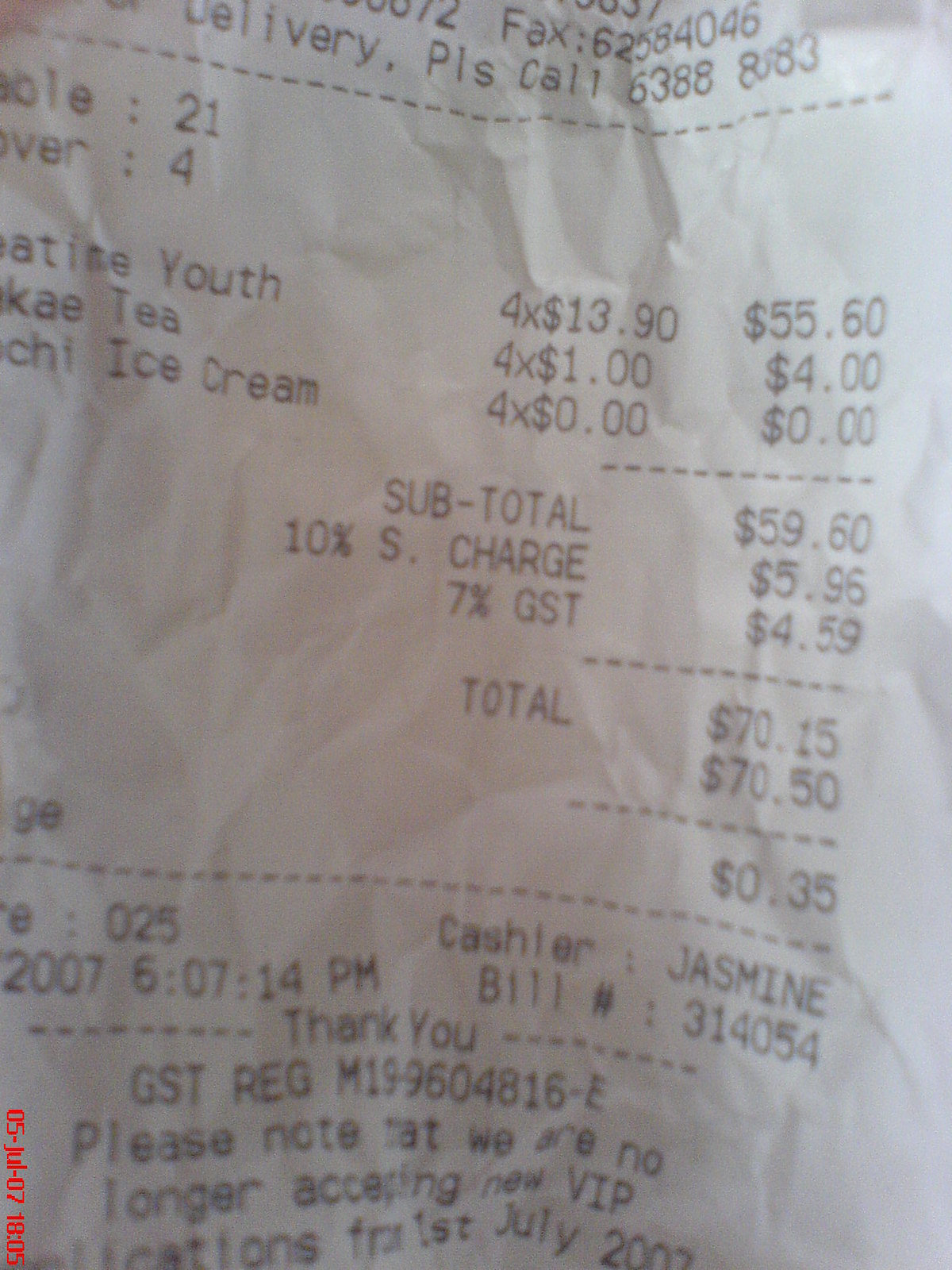This is a detailed close-up photograph of a slightly wrinkled white receipt with black text and numbers, partially cut off on the left side. The receipt features several key details: on the bottom left, written sideways in red, is the text "05-July-07-18-summer-colon-05". At the top, the receipt displays the numbers "FACTS-62584046" and "DELIVERY-63888383" followed by the numbers "21" and "4". Below, the receipt lists items such as "YOUTH", "TEA", "ICE CREAM" and "4X". Further down, complex pricing details include subtotal $59.60, 10% tax of $5.96, and 7% GST of $4.59, totaling $70.15, with $70.50 tendered, providing a change of 35 cents. The date, "2007", with a timestamp of "14 seconds after 6.07 p.m.", is also mentioned. The cashier’s name was Jasmine, and the bill number is 314054. A note indicates that VIP applications were no longer accepted from July 1, 2007. The receipt concludes with a "thank you" and additional instructions, though the store name is not visible.